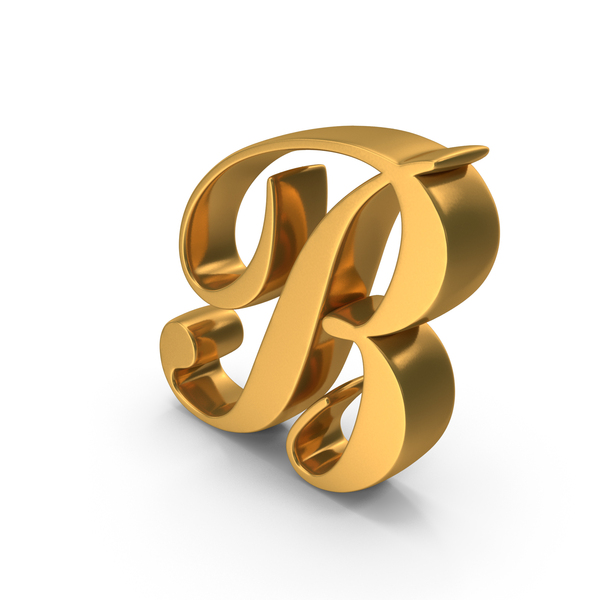The image showcases a digitally produced, three-dimensional, uppercase letter 'B,' rendered in a fancy cursive style. The 'B' is gold and visibly reflective, giving it a metallic appearance. This golden 'B' features intricate swoops and curls, highlighted by varying shades of gold that emphasize its dimensionality and the play of light across its surfaces. The front face of the letter is a solid, bright gold, while the sides and shadowed areas have a darker gold hue, enhancing the overall depth. Positioned at an angle, it appears as if it were tilted to the four o'clock position, providing a dynamic and elegant perspective.